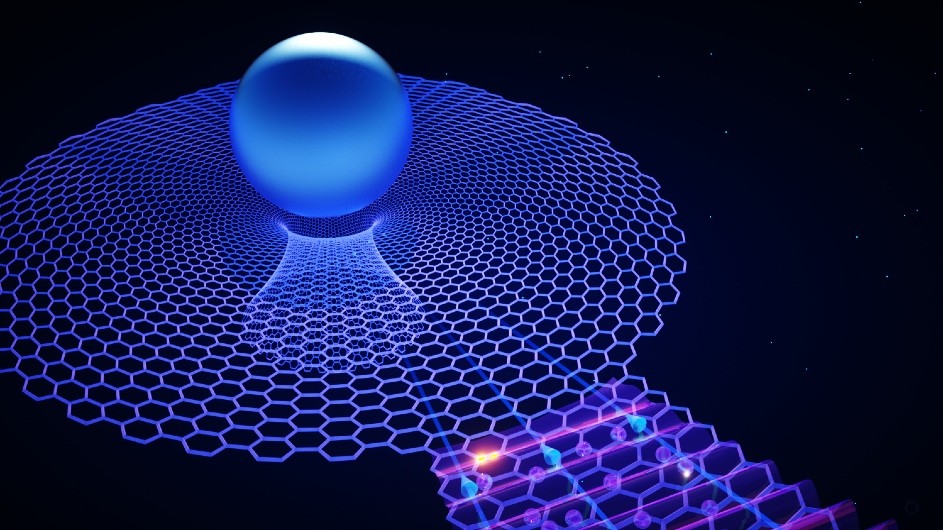The image depicts a computer-generated, three-dimensional scene set against a black background reminiscent of the depths of space. At its center, a striking blue sphere is encased in a honeycomb pattern of interconnected hexagons, forming a circular enclosure around it. Below this encircling pattern, the honeycomb structure extends downward, creating a walkway leading to the central sphere. Intricate lighting, featuring hues of blue and purple, enhances the visual complexity and ethereal quality of the image. The sphere casts a subtle shadow, adding to the depth and realism of the scene, which evokes a futuristic, otherworldly atmosphere.